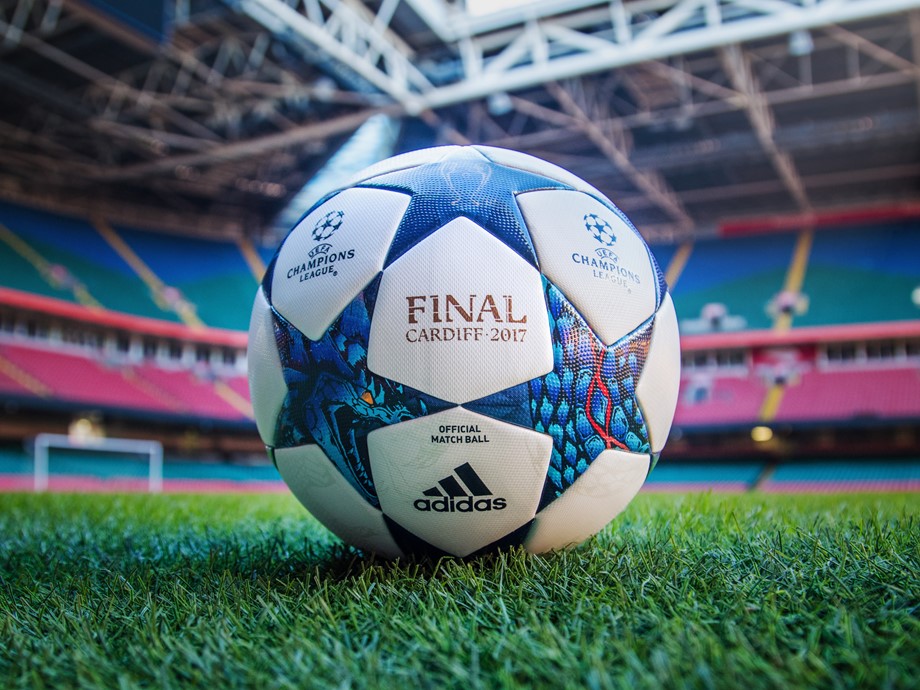The image depicts a close-up of an Adidas soccer ball placed centrally on a lush green grass pitch. The ball prominently features various inscriptions and logos. At the bottom front section of the ball, "Official Match Ball" is printed in black against a white shield-shaped outline. Directly below this, the Adidas logo and symbol are visible. In the middle of the ball, "Final Cardiff 2017" is displayed in gold letters within a white shield outline set against a blue background. Adjacent to this, there are blue stars with intricate patterns incorporating light blue and dark blue hues, some accompanied by red streaks. The Champions League logo appears in black on a white background on both the upper left and right sections of the ball. The ball is beautifully textured, showcasing fine dots across its surface.

In the backdrop, an expansive domed stadium envelops the scene. The stadium features empty stands decked out in a gradient of colors, with purples and blues transitioning up to the ceiling. A net is faintly visible beneath the stands, adding depth to the setting. The overall scene captures a moment of solitude and anticipation, the ball laying in wait on the perfectly manicured grass.